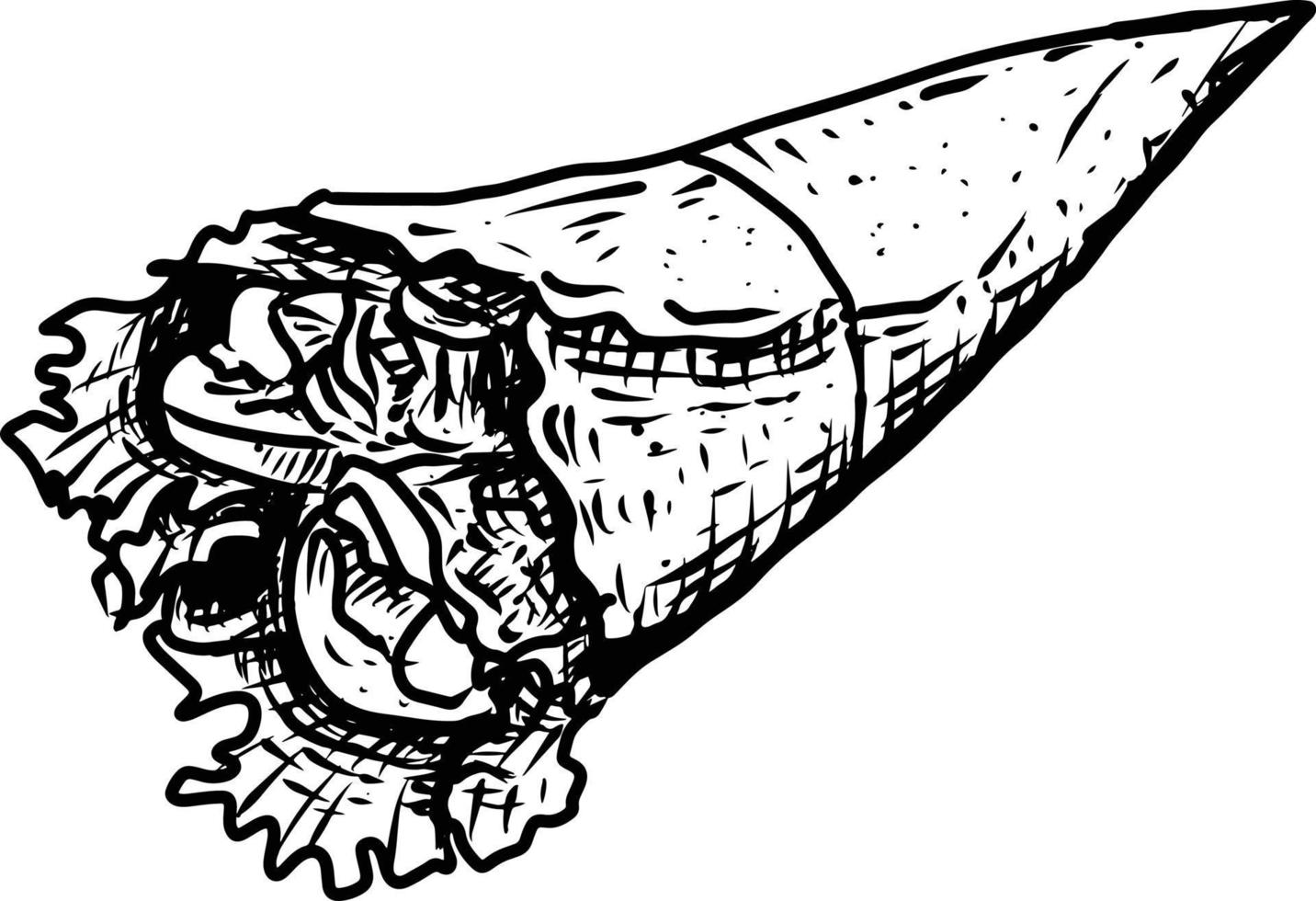This black-and-white illustrated image, resembling a piece of abstract clipart, depicts a cone-shaped object. The narrowest point of the cone is situated at the top right, widening towards the bottom left. Though the image is drawn with thick, heavy black lines, it remains unclear whether the object represents a type of food like a sandwich or something else, such as a bouquet of flowers. The exterior of the cone-like structure looks rough, marked with lines, dots, and patchwork patterns. Inside the cone, visible at the wider opening on the left side, are indistinct objects, possibly food or fruit, further obscured by dark, dense lines. An additional detail includes what appears to be tissue paper or a wrapper protruding from the bottom left, adding to the overall messiness of the design. The entire composition is rendered without shading, purely in black lines against a stark white background, enhancing its abstract and enigmatic nature.